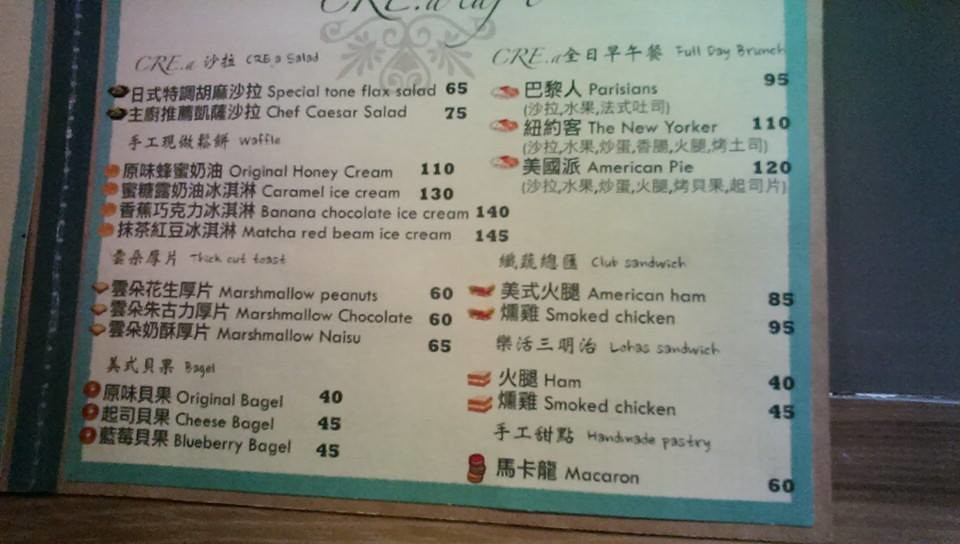The image showcases a bilingual menu with both Chinese and English text, alongside listed prices. At the top of the menu, the restaurant name appears truncated and is not fully visible. The menu begins with an item labeled "CRE, CRE, Salad" in English, accompanied by a Chinese description, and lists "Special Tone Flax Seed Flax Salad" priced at $65.

Following this, another salad option is presented with the Chinese name and its English translation, "Chef Caesar Salad," priced at $75. Next on the menu is the Chinese term for "Waffle," followed by the English word "Waffle." This section includes four varieties:

- Original Honey Cream Waffle at $110
- Caramel Ice Cream Waffle at $130
- Banana Chocolate Ice Cream Waffle at $140
- Matcha Red Bean Ice Cream Waffle at $145

The next category is "Thick Cut Toast," listed with its Chinese equivalent and the following variations:

- Marshmallow Peanuts Toast
- Marshmallow Chocolate Toast
- Marshmallow Naisu Toast

The menu then features a selection of bagels, again listed with their Chinese names:

- Original Bagel
- Cheese Bagel
- Blueberry Bagel

Additionally, the menu offers full brunch options, identified by their descriptive names in English:

- New Yorker
- American Pie
- American Ham
- Smoked Chicken Sandwich
- Ham Sandwich

Finally, the menu concludes with an item labeled "Macaroon" with its corresponding Chinese translation.